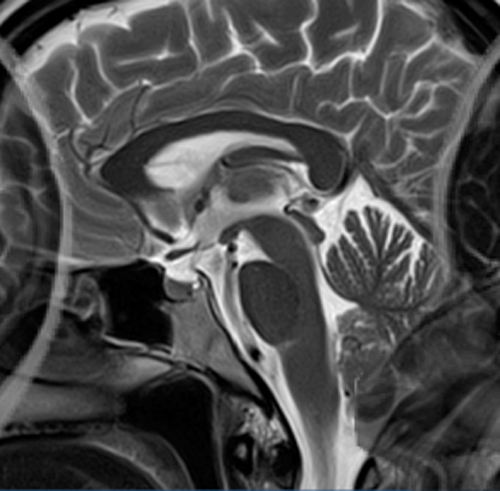This image resembles an x-ray or medical scan of a brain shown in black and white. The brain, viewed in a cross-sectional side profile, reveals intricate details including the wrinkly nodules of the brain mass and branching vessels. The cerebellum, hypothalamus, and both gray and white matter are discernible, despite the overall slight blurriness or lack of focus. The image also features a stem-like structure in the middle and gives the impression of additional, less identifiable structures or shadows. Some areas of the image, particularly the left and right sides, appear distorted, possibly by a clear overlay. The abstract quality of the design introduces elements that resemble plant-like parts or even a distorted face, contributing to its unique, almost artistic appearance.